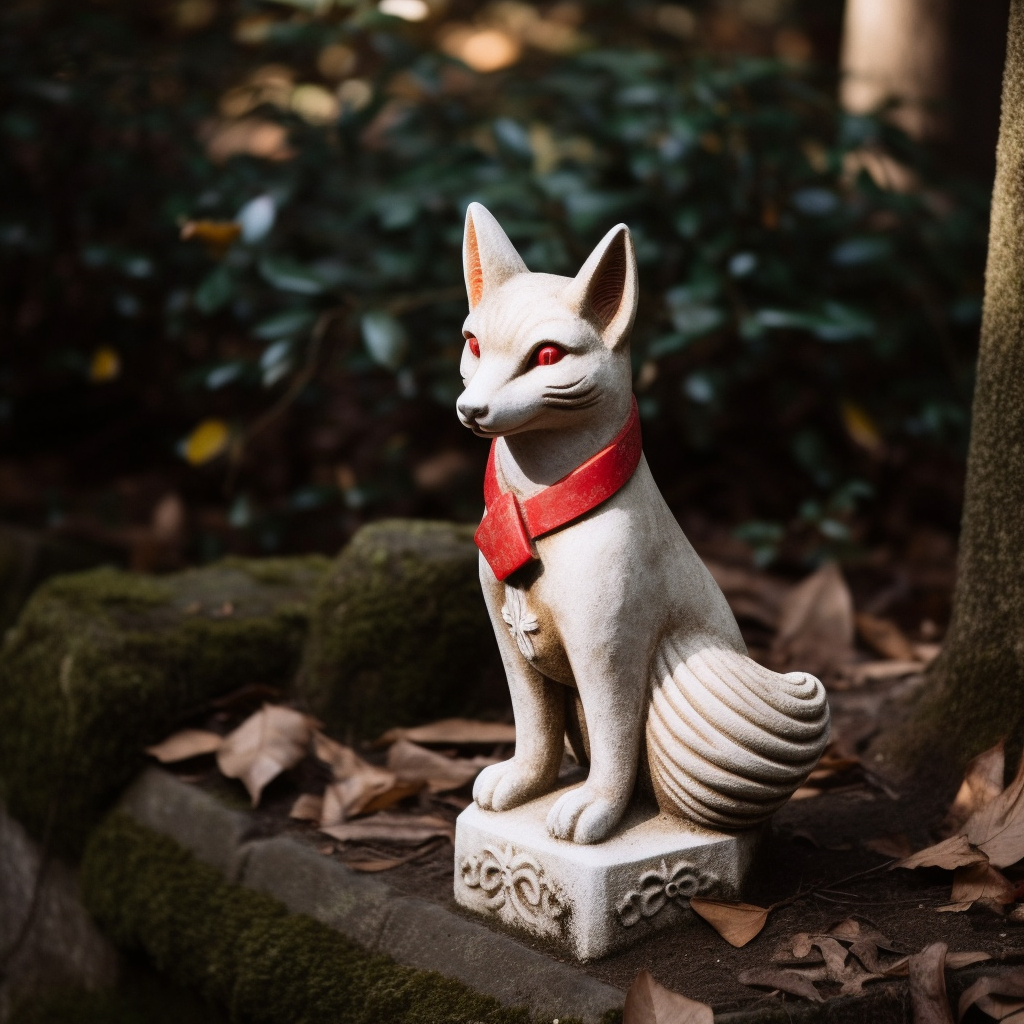The image showcases a small, white statue of a fox with piercing red eyes and orange ears, tied with a red ribbon around its neck. The fox sits on a square base in a garden, its fluffy tail curled prominently to the side. Its front paws stretch forward, and it has an alert posture, seemingly due to its wide-open red eyes. The garden environment includes a gray stone surface with dark brown dirt, partially covered by moss. The background features blurry dark green leaves, a large green bush, a tree trunk to the right, and dead leaves scattered on the ground.